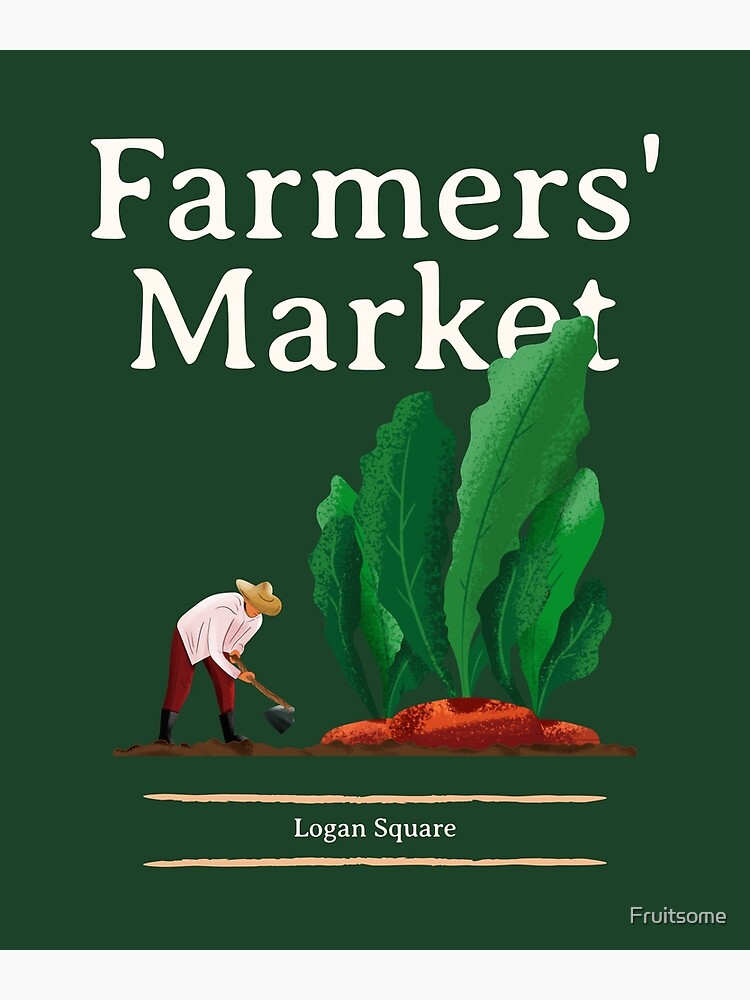The image appears to be a computer-generated logo or marketing flyer for a farmer's market, dominated by a green background. At the top, a white banner spans the width of the flyer. Below this banner, large white letters prominently display the text "Farmer's Market." Situated underneath this text is a detailed illustration featuring a farmer tending to a garden on the left side, with a hoe in hand. On the right side of the image, green leaves and red beets protrude visibly from the ground, with a small patch of dirt beneath them. At the bottom of the flyer, there is a narrow white border. In small white letters within this border, the text "Logan Square" is neatly printed. Additionally, "Fruitsome" is written in white text in the lower right corner of the flyer. The entire flyer measures approximately eight and a half by eleven inches.